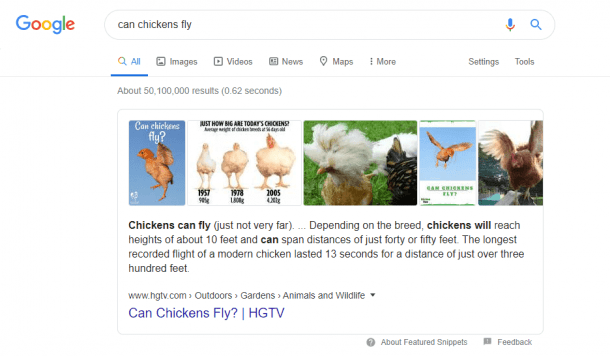A Google search page is depicted, showcasing the vibrant Google logo with its iconic blue, red, yellow, and green letters. Below the search bar, where the query "Can Chickens Fly?" is typed, a variety of related images appear. 

1. The first image features a small chick framed within a blue square, titled "Can Chickens Fly?" 
2. The second image addresses "Just How Big Are Tommy's Chickens?" and illustrates three chickens of different sizes, compared over the years 1957, 1978, and 2005.
3. Following this is an image of several chickens nestled in lush green grass.
4. Another image shows a chicken soaring through a clear blue sky.
5. Lastly, there's a picture of a chicken on the ground, mid-flutter, accompanied by text that reads: "Chickens Can Fly, Just Not Very Far. Depending on the breed, chickens will reach heights of about 10 feet and can span distances of just 40 or 50 feet. The longest recorded flight of a modern chicken lasts 13 seconds for a distance of just over 300 feet."

Beneath these images, a green-highlighted section with the header "Can Chickens Fly?" appears, followed by a line and the logo for HGTV.